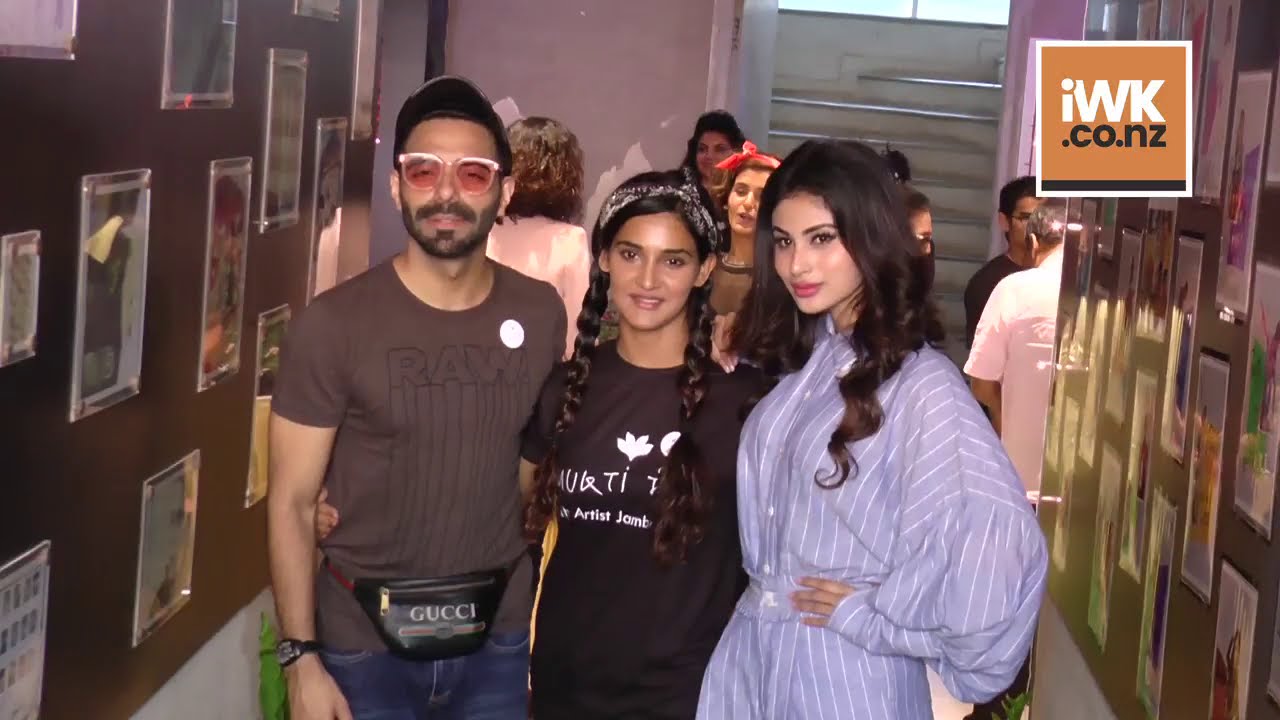In this image, we see a vibrant setting that resembles a gallery or house party with a bustling atmosphere marked by various people milling around. The focal point is three individuals standing together, posing for a photograph, positioned centrally in the hallway framed by brown walls adorned with framed pictures. 

On the left is a man with short dark hair and a beard, donning a tight brown t-shirt emblazoned with the word "RAW" in black letters. He accessorizes with white-framed sunglasses, a black Gucci fanny pack with a gold zipper, and a black band on his right wrist, paired with blue jeans. 

In the middle stands a young woman, likely in her twenties, smiling cheerfully. She has long dark hair styled in braids that fall over her shoulders and wears a headband. Her attire consists of a brown t-shirt with possibly some white detailing. 

On the right, a woman with long dark hair cascading past her shoulders is seen in a light blue and white striped outfit that appears to be a romper. She exudes a youthful and model-like presence. 

The backdrop features people and possibly more framed photos. A staircase bends to the right, with natural light pouring in, visible at mid-landing. The top right corner of the image displays a logo "iwk.co.nz" on an orange background, indicating a possible website. The entire scene radiates a lively, social ambiance with intricate details throughout.